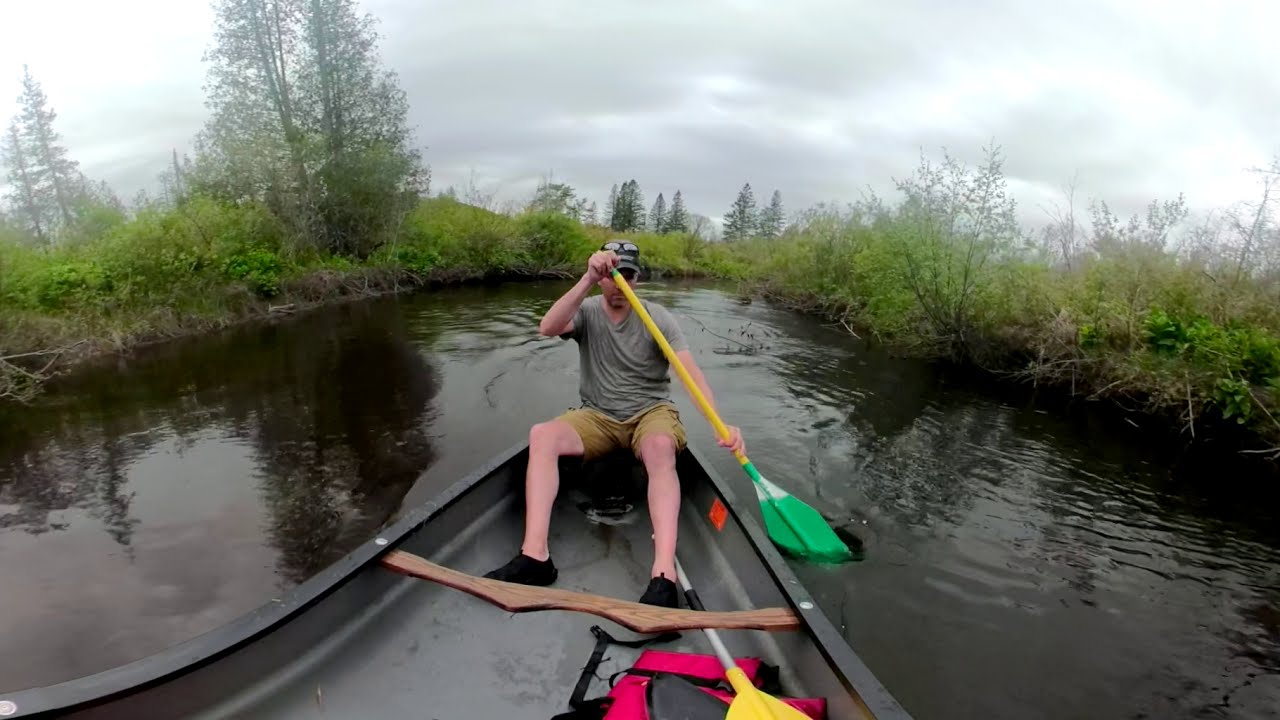The photograph captures a thin man in his 40s, seated at the back of a dark gray, two-person canoe. The man, focused on paddling, wields a distinctive paddle with a yellow shaft and a green blade that is partially dipped in the black, reflective water of a calm river. His face is partially obscured by the paddle as he rows. He is dressed in a gray t-shirt, light brown shorts, black shoes, and a baseball cap adorned with sunglasses. Inside the canoe, there is also a red life vest with black straps and a second paddle at the bottom. The river is surrounded by dense greenery, consisting of brambles, bushes, and a few trees that break up the landscape. The overcast sky above is filled with gray clouds, adding to the serene yet somber atmosphere of the scene.